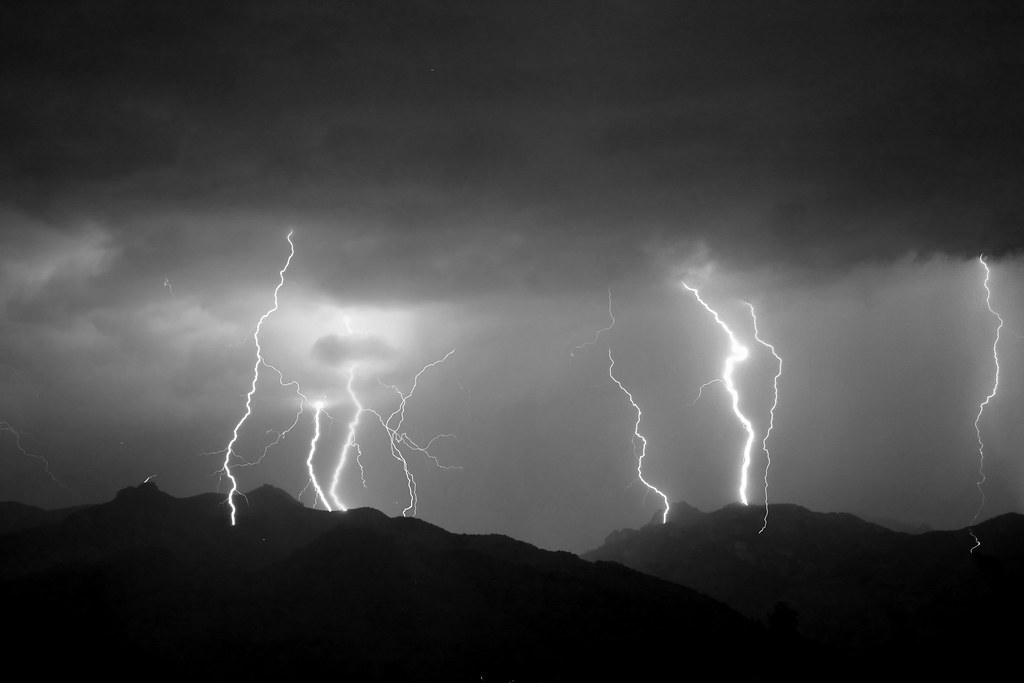In this striking black-and-white photograph, a dramatic nighttime thunderstorm dominates the scene with a sky that transitions from pitch black at the top to a dark grey towards the bottom. The tempestuous clouds appear nearly black, hinting at the ferocity of the impending storm. Below the turbulent sky, a rugged landscape of mountains stretches across the horizon, shrouded in shadows and dim light. Numerous bolts of lightning—at least seven to nine—crash down from the sky, illuminating the clouds and striking various points on the mountains. The lightning bolts vary in size and intensity, with some thin and solitary while others are larger and more brilliant. The eerie stillness of the grey, foggy middle ground between the mountains and the stormy sky enhances the sense of awe and fear. The stark contrast and high drama of the scene make it a mesmerizing and somewhat frightening capture of nature's raw power.